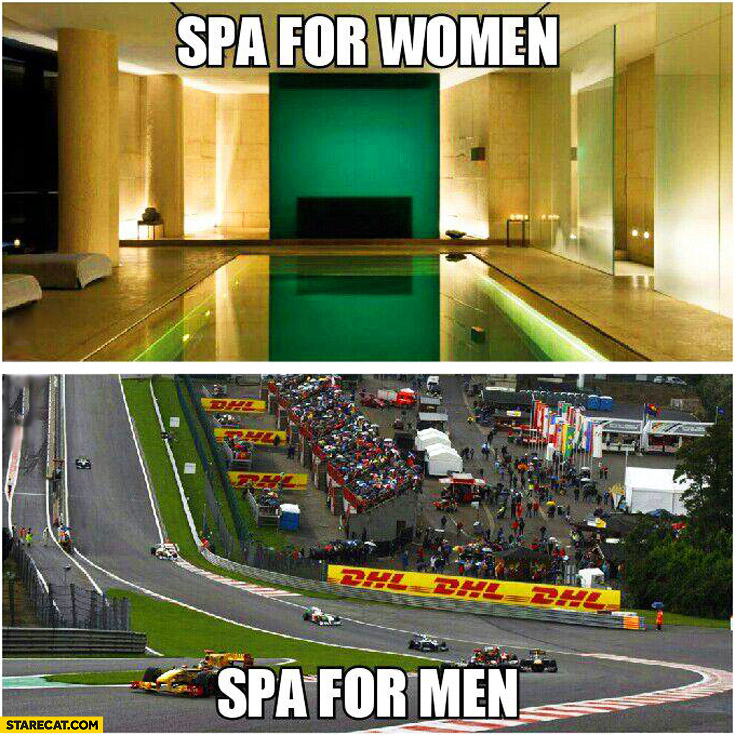The image is a humorous meme split into two sections to highlight gender stereotypes regarding relaxation preferences. The top half, labeled in large white letters as "Spa for Women," showcases an opulent indoor spa. This setting features a serene, luxurious infinity pool with soft lighting emanating from golden-hued stone walls and glass sliding doors. Lounge beds line the sides, making it a quintessential place for peaceful indulgence. A green wall in the background adds a calming touch. In contrast, the bottom half, captioned "Spa for Men" in white letters, depicts a bustling racetrack. Here, race cars zoom along the track, surrounded by spectators and numerous DHL advertisements in red and yellow. This energetic scene suggests that men relax by immersing themselves in high-octane activities. The website "StareCat.com" is noted in dark lettering within a yellow box in the lower left corner, indicating the source of these juxtaposed images.